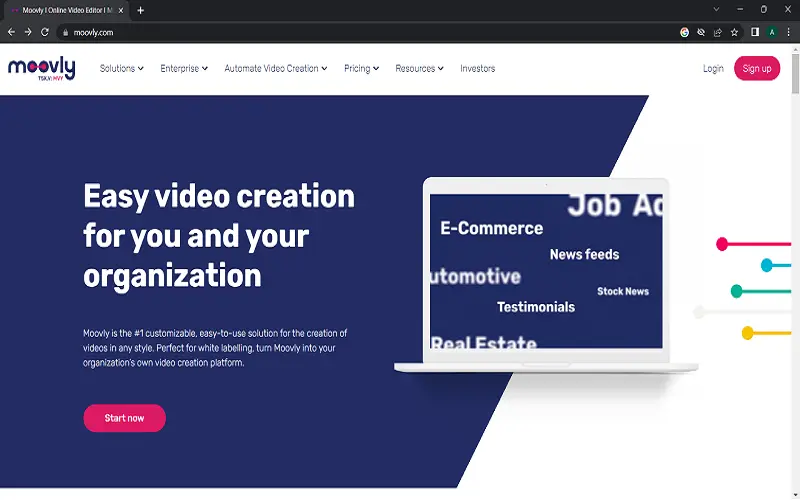This is a detailed screenshot of the Movely website. The URL bar clearly displays "movely.com," indicating the active webpage. In the top-left corner, the Movely logo is prominently featured. The logo showcases the word "Movely" in blue against a white background, with a unique design element where the letter 'O’s are connected by a pink line running through the center of the circles.

Adjacent to the logo, there are six navigation tabs written in blue text: "Solutions," "Enterprise," "Automate Video Creation," "Pricing," "Resources," and "Investors." Moving to the top-right corner, the website provides a pink "Sign Up" button and a "Login" tab for user access.

The central part of the site features a large trapezoid shape that covers approximately 70% of the screen. Inside this trapezoid, there is large white text displaying the message, "Easy Video Creation for you and your organization." Finally, towards the bottom of the trapezoid, there is a "Start Now" button in pink, inviting users to begin their journey with Movely.